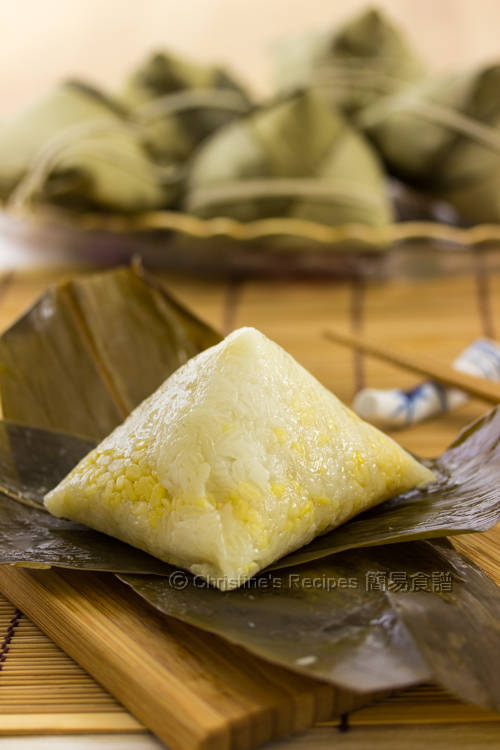This is a detailed photograph showcasing a steamed bun with a white, doughy exterior featuring a hint of yellow. The bun sits atop what appears to be leafy wraps, possibly seaweed or another type of leaf, placed on a wooden board set against a bamboo sushi rolling mat. In the background, a plate with five or six similar buns wrapped neatly in leaves and tied with string can be seen. These background buns are slightly out of focus, enhancing the prominence of the foreground bun. Additionally, a pair of chopsticks rests on a white and blue holder towards the back right of the scene. The overall color palette of the image includes tones of white, yellow, green, and brown. The watermark in the corner credits "Christine's recipes."